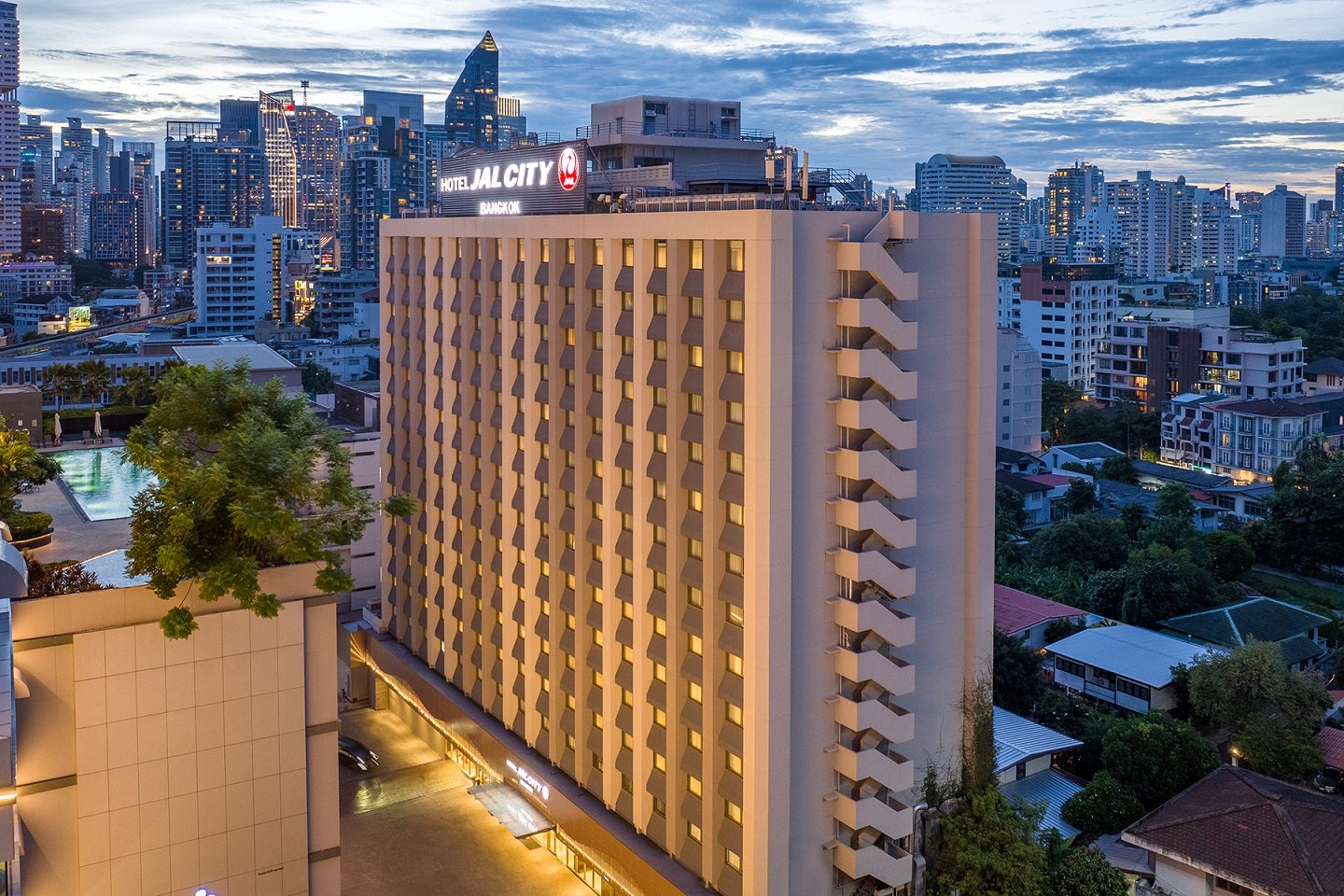This vibrant photograph captures a dynamic cityscape in Bangkok with an emphasis on the towering Hotel JAL City Bangkok, highlighted by its distinctive architectural features and vibrant surroundings. The hotel's asymmetrical appearance dominates the frame, with its right side appearing larger due to the diagonal tilt of the structure. This tall building, reaching at least 15 floors, is adorned with numerous small, glowing yellow windows that add a warm ambiance to the scene. One notable feature is an exterior staircase on the right, climbing up to the roof.

The hotel's name, "Hotel JAL City Bangkok," is prominently displayed on a wide rectangular board in bright white letters at the top. The sign also features a logo with a red and white circle containing a red bird and the letters "J-A-L."

Adjacent to the hotel on the left bottom corner, there is a beige building featuring a green rooftop interspersed with trees and a light blue swimming pool. In the backdrop, the cityscape is rich with several high-rise buildings, their lights piercing the dusk. The sky is a darkish blue, adorned with white clouds, suggesting the onset of evening. The overall city view, complemented by the interplay of lights and architectural elements, vividly illustrates the bustling yet serene essence of downtown Bangkok.